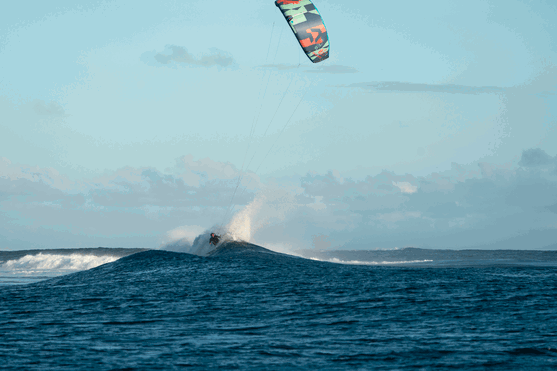The image captures an exhilarating scene of a parasurfer in the middle of the ocean, emphasizing the grandeur and isolation of the setting. The parasurfer, dressed in a black wetsuit, navigates through small, cresting waves topped with white splashes. The grandeur of the open sea is accentuated by the absence of visible land and the minuscule appearance of the surfer, highlighting the scale and extremity of the activity. The parasail, colored with a black background adorned with orange and mint green shapes, soars high in the sky, tethered to the surfer below. The sky itself is a gradient from light to dark blue, dotted with puffy white clouds. Positioned slightly off-center to the left, the parasurfer becomes the focal point against the expansive, dark blue ocean and the vibrant, kite-like sail. The photograph, taken in the daytime, masterfully encapsulates the thrill and vastness of parasurfing amidst an endless marine backdrop.